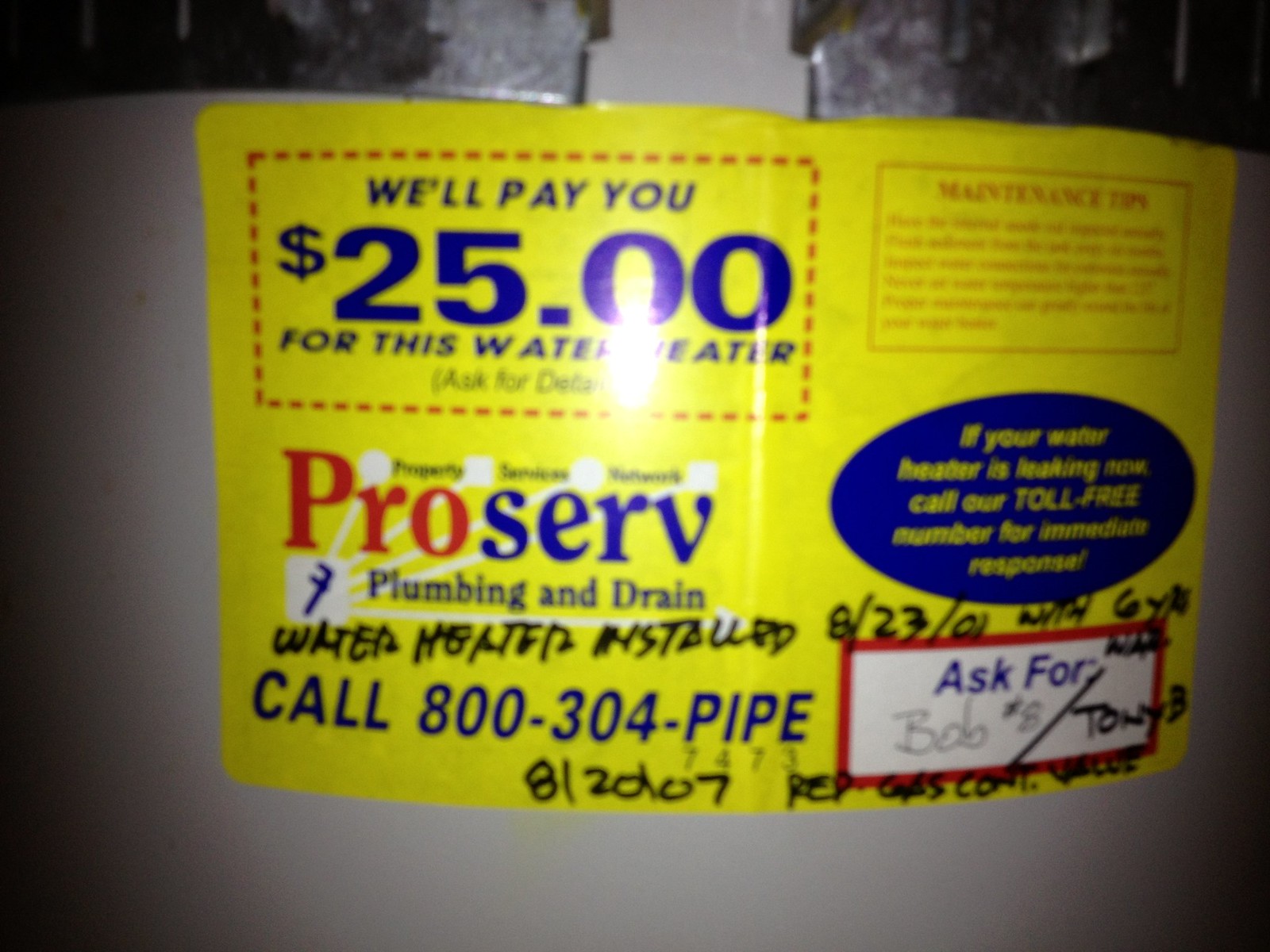In a dimly lit basement, a close-up photograph captures a white, curved water heater, adorned with brackets and metallic fittings on its top. A prominent yellow sticker is affixed to the heater, featuring bold colored text and various annotations. At the top of the sticker, a red dotted rectangle frames blue text offering, "We'll pay you $25 for this water heater," with a note in parentheses urging, "Ask for details." Below this message is the logo "ProServe Plumbing and Drain," accompanied by additional branding text: "ProServe Property Services Network."

Handwritten with a sharpie are the words, "Water heater installed 8-27-01," albeit accompanied by some unreadable marks. The sticker also instructs, "Ask for Bob or Tony," and provides a toll-free number, 800-304-PIPE, surrounded by a blue circle with yellow text indicating to call immediately if the water heater is leaking. A square with a red border on the right side of the sticker mentions "Maintenance Tips," but the finer details are too blurry to decipher.